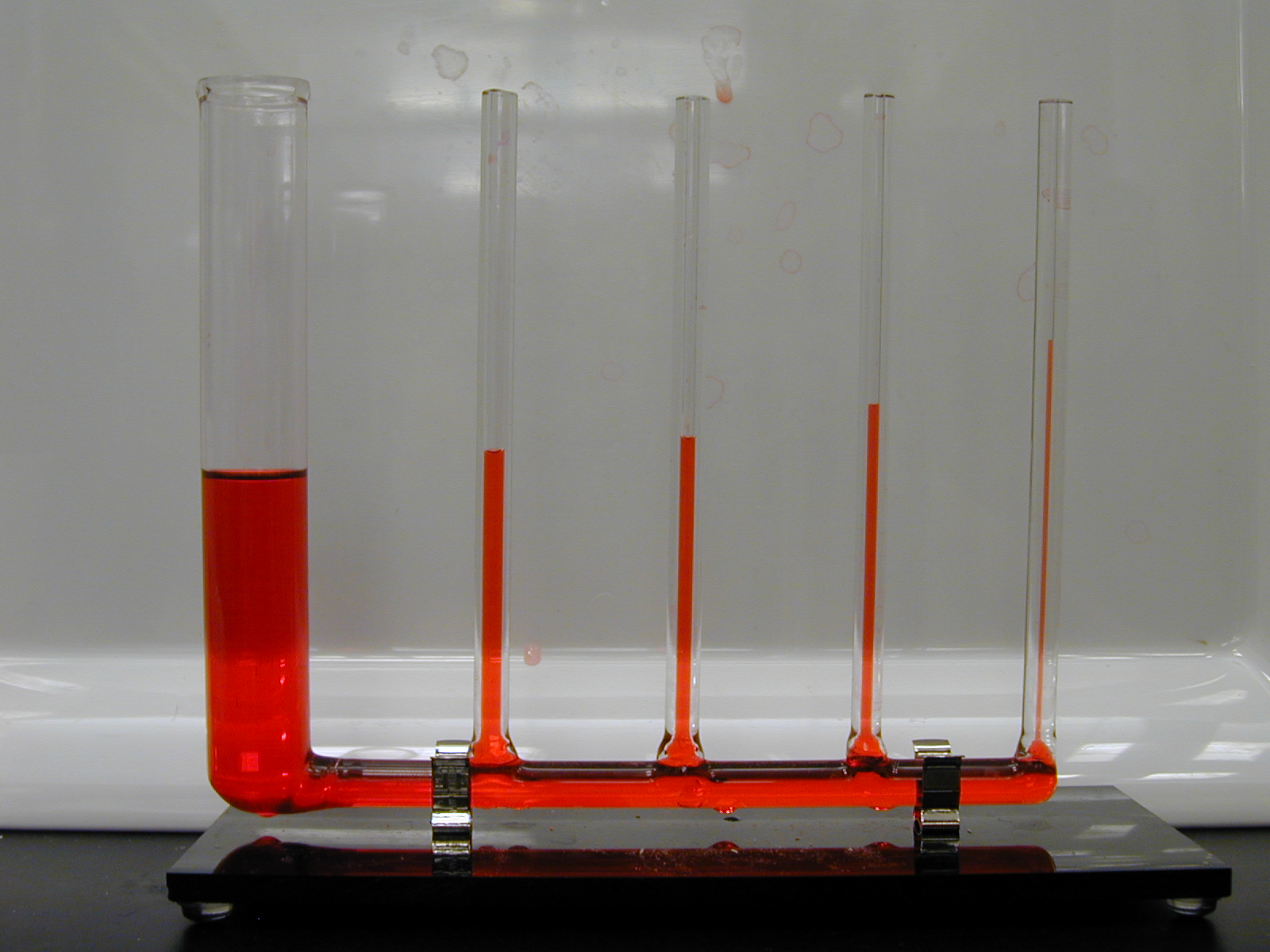The image depicts a scientific measuring instrument set in a laboratory environment. At the center of the composition is a beaker-like apparatus with a series of connected test tubes, five in total, arranged from left to right. The largest tube is on the left, gradually decreasing in size to the smallest on the right. Each tube contains a reddish-orange liquid, with the volume decreasing from left to right, creating a gradient effect. The entire setup is supported by a metal clamp attached to a flat, oblong base with small glass legs. The background features a shiny, white porcelain-like wall, and the apparatus rests on a dark, black surface, contributing to the contrast of the scene.